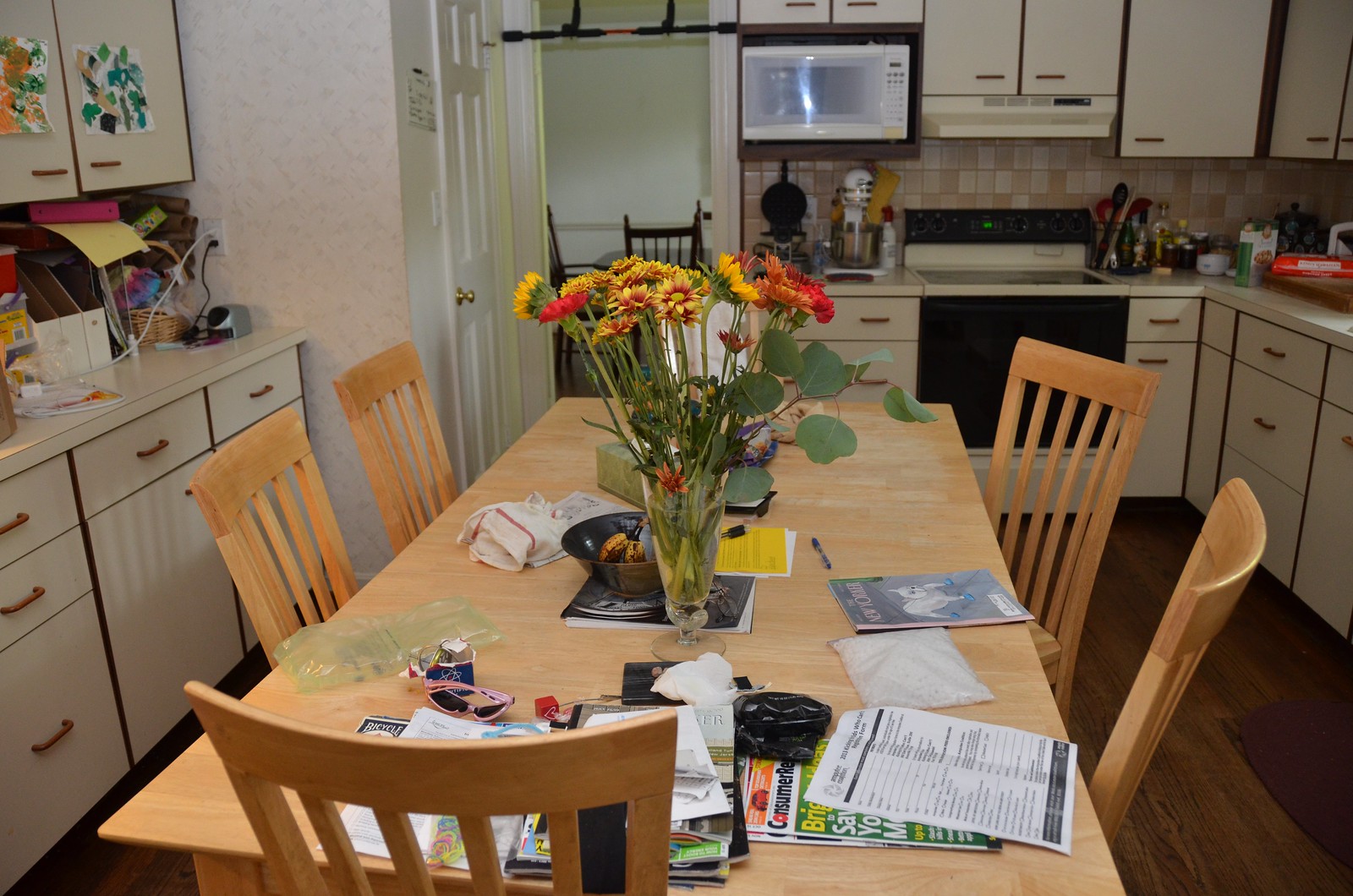The image depicts a typical American kitchen that exudes a well-used and lived-in feel. Central to the scene is a kitchen table made of white oak, surrounded by six chairs. The proximity of the kitchen cabinets, microwave, and sink to the table suggests that the dining area is integrated into the kitchen space. The countertops and kitchen table are cluttered with various items, giving the room a busy atmosphere. On the table sits a vase of flowers alongside some half-eaten food, a Consumer Reports magazine, a New Yorker magazine, assorted mail, papers, and even a pair of sunglasses. Evidence of a recent package delivery is visible, with protective packaging material scattered around. The presence of children's finger paintings and colorful artwork on the cabinet doors indicates that this is a family home with young children. Overall, the kitchen is filled with signs of active daily life, showcasing the dynamic environment of a household deeply engaged in its living space.